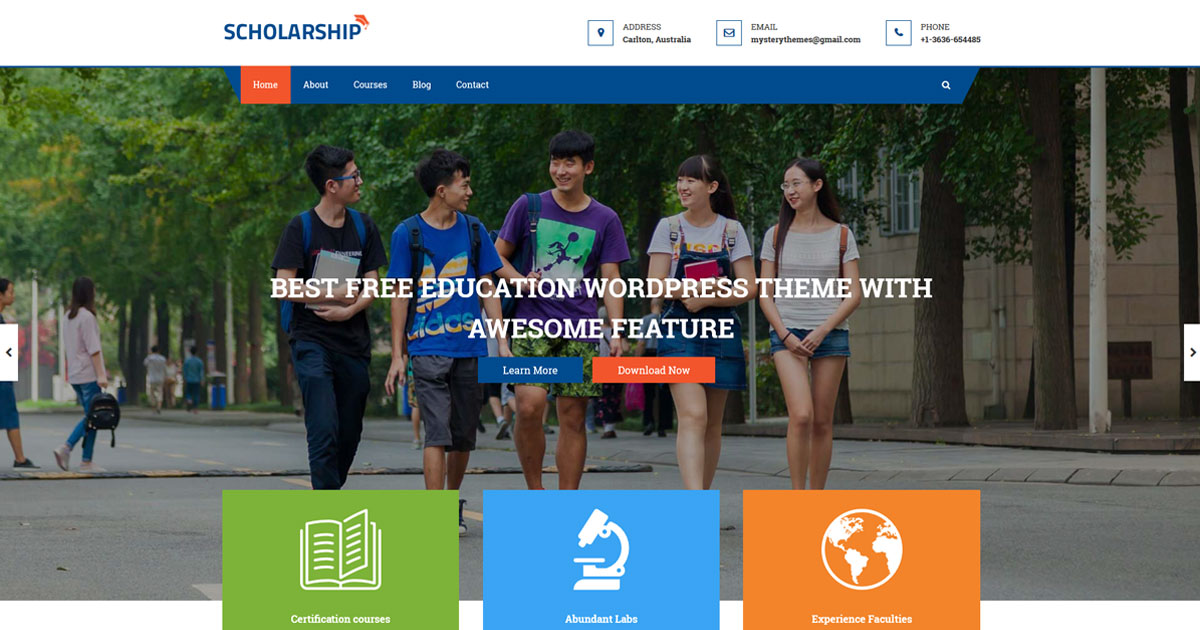**Website Screenshot Description:**

The screenshot captures a section of a website focused on scholarships and education. In the upper left corner, the website's logo features the word "Scholarship" in blue lettering with an orange graduation cap icon beside it. To the right of the logo, contact information is partially visible, suggesting a location in Australia with icons for email (a Gmail address) and a phone number, though the exact details are unreadable.

A blue header bar spans the top of the page, containing navigation links labeled Home, About, Courses, Blog, and Contact. The Home button is highlighted in orange, indicating the current page selection. Below the header, a prominent image showcases five students, presumably of Asian descent with short black hair, walking towards the camera. The two male students on the left are dressed casually, one in jeans and the other in shorts with graphic tees. The two female students on the right wear short skirts, also moving forward with a casual demeanor.

The image bears an overlay text promoting the website's theme: "Best Free Education WordPress Theme with Awesome Features." Two call-to-action buttons are present below the text: a blue "Learn More" button on the left and an orange "Download Now" button on the right.

Further down the page, there are three informational panels:
1. **Certification Courses:** A green panel with a white open book icon.
2. **Abundant Labs:** A light blue panel with a white magnifying glass icon.
3. **Experience Faculties:** An orange panel featuring a white globe icon with geographic markings.

Each panel offers more details about the respective features or services provided by the website.